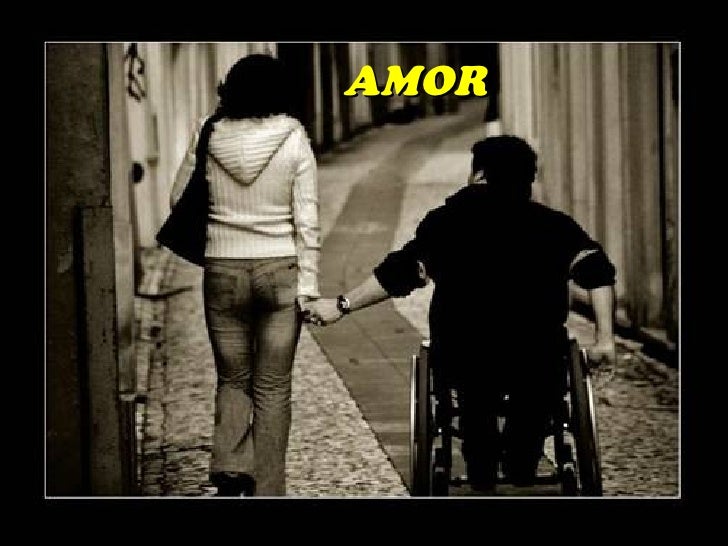In a pixelated, monochrome brown photograph framed with a thin black and white border, two individuals are depicted from behind as they navigate a narrow European-style alley or corridor. On the left, a woman with dark hair is dressed in a white hoodie, blue jeans, and holds a black purse in her left arm. She walks beside a man in a wheelchair, who is wearing a black hoodie and black jeans, also featuring a watch on his wrist. The man looks up at the woman as they hold hands. Above their heads, in large yellow capitalized letters, the word "AMORE" is displayed. The image, though not of high quality, evokes a sense of companionship and shared journey.